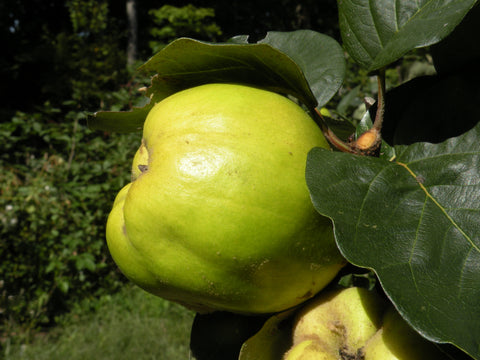This photograph captures a stunning green apple bathed in natural sunlight, prominently positioned in the center against a leafy backdrop. The light green apple, reflecting a bright white light as though sunshine is directly hitting it, is surrounded by lush dark green waxy leaves. To the right and partially underneath the main apple, a smaller, less vibrant green fruit with some brown fuzz is visible. The top right corner of the image is filled with more waxy leaves, while in the background to the left, green bushes and leafy branches add depth to the scene. Tiny white flower buds can also be seen amidst the foliage, suggesting growth and the promise of new blooms. The overall impression is one of vibrant nature, caught in a moment of serene daylight.